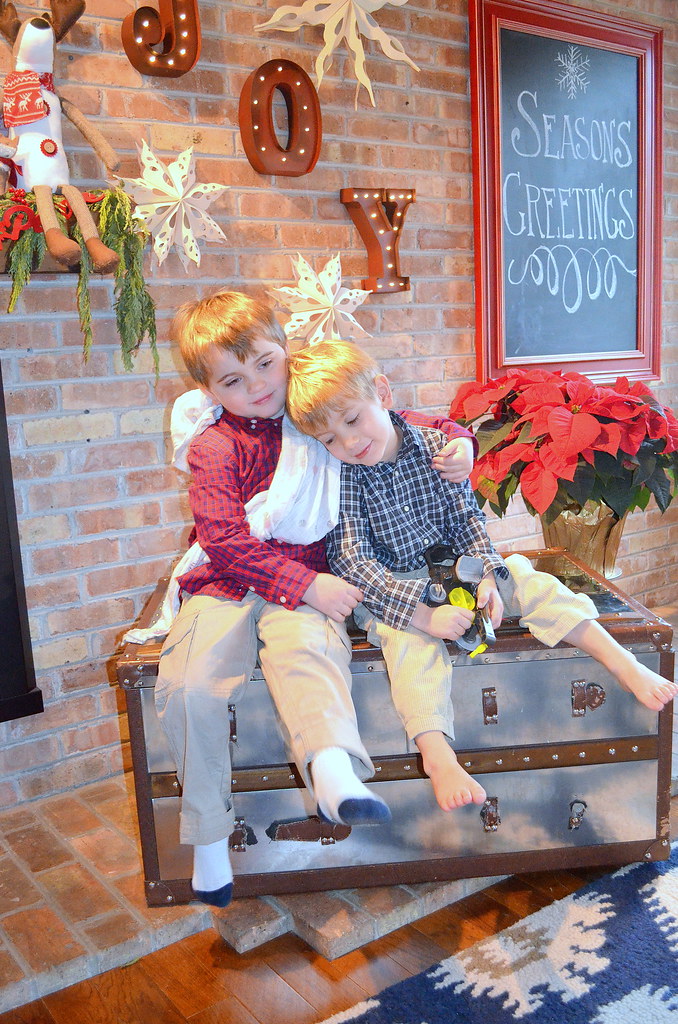The photograph depicts a heartwarming Christmas scene featuring two young red-haired boys sitting on a large trunk with a silver front and wooden borders. The older boy, dressed in a red and black checkered shirt with beige pants, has his arm lovingly wrapped around his younger brother, who is wearing a black and white checkered shirt with matching beige pants and no socks. Their setting includes a hardwood floor adorned with a blue and white carpet. Behind them, a red brick wall is festively decorated. To their left, large illuminated letters spelling "JOY" hang diagonally with tiny lights. A poinsettia in a gold foil-lined pot adds a touch of seasonal cheer, while a shelf above holds a stuffed reindeer with thick antlers and a scarf. To the right, a red-trimmed blackboard chalkboard inscribed with "Season's Greetings" is accented with a snowflake. The boys' affectionate pose captures a tender sibling moment amidst the festive decorations, evoking the warmth and joy of the holiday season.